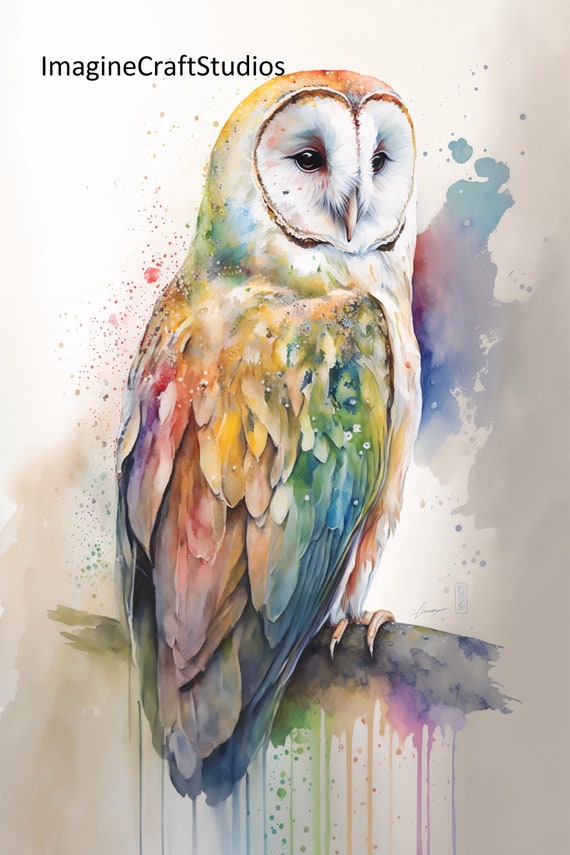This image portrays a contemporary, graphic watercolor painting of an owl, possibly AI-generated due to some inconsistencies. The artwork is by Imagecraft Studios, as indicated by the black text at the top of the image. The owl, eye-catchingly adorned in a spectrum of rainbow colors—yellows, greens, blues, oranges, reds, purples, and pinks—stands out against a textured background with paint splotches and drips extending down the canvas. Each feather is intricately detailed in its own hue, contributing to the vivid mosaic. The owl is positioned with its back facing the viewer, but its head is turned so that its dark eyes and brownish beak are visible. The face is white, with delicate strokes that highlight the feathered texture. Perched on a tree limb at the bottom of the image, the owl's talons gripping the branch are depicted, albeit with some anatomical inaccuracies that suggest the possibility of AI generation. The overall depiction combines realism with a whimsical, multicolored aesthetic, making the owl appear both cute and mesmerizing.